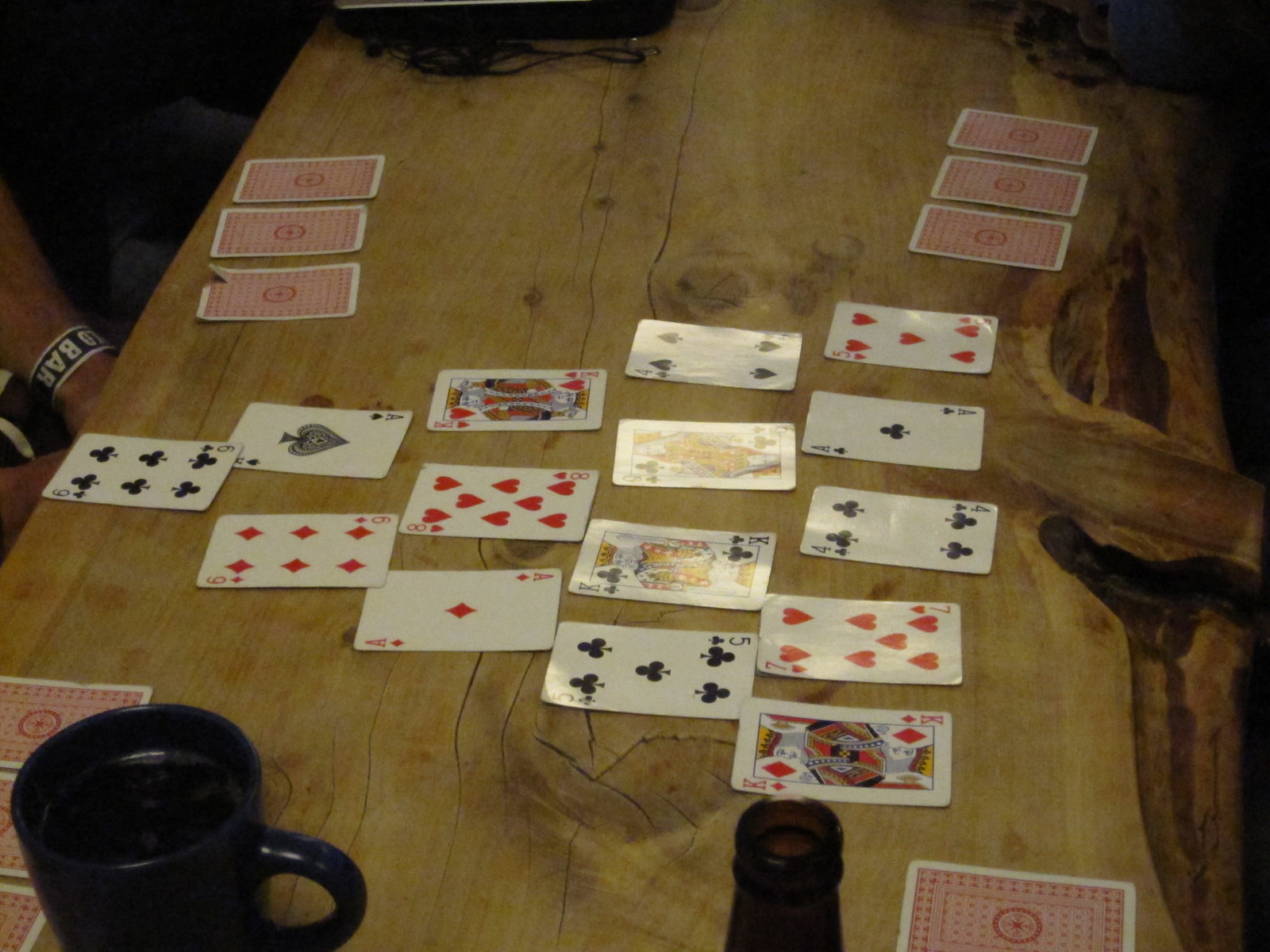The image captures a lively scene at a convivial gathering, centered around a wooden table where a card game is underway. The table, made from light-grain wood, dominates the frame with its natural beauty highlighted by knots, lines, and various shades of brown running from the bottom to the top of the image. To the left edge of the table, a portion of an arm is barely visible, its light skin adorned with a black and white graphic bracelet. 

A dark blue or black coffee cup sits in the bottom left corner, filled with what appears to be black coffee or tea. To the right of the cup, the neck of a dark brown beer bottle peers into view, its cap removed. 

The card game sprawls across the table. On the left side, three cards are laid face down, with another set of three cards further toward the coffee cup. These cards share a consistent design: a white border framing a red square and a central circle. On the right side, three more face-down cards appear, with a single card further down at the bottom right of the image. 

In the middle of the table, an engaging array of face-up cards forms a pyramid-like structure, starting with five cards in the top row and reducing by one card per row to a single card at the bottom. Visible cards include the Queen, Seven of Hearts, Four of Clubs, Ace of Spades, and various Kings and Queens from different suits. The vibrant mix of reds, blacks, and intricate patterns from the cards enhances the sense of camaraderie and engagement around the table.